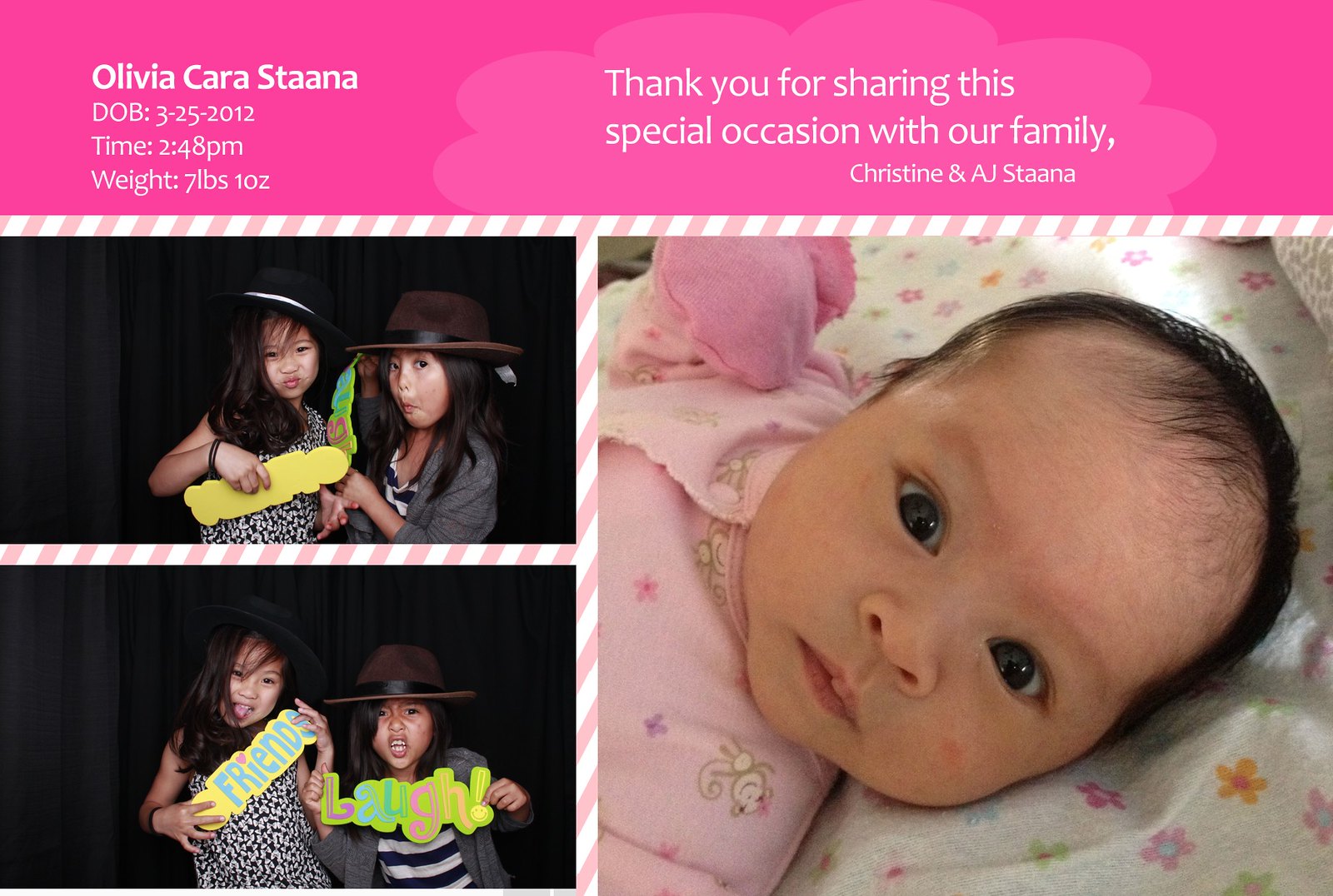This wide rectangular card features a bright pink banner across the top with a tiny lighter pink cloud on the right side. In bold white font on the left, it reads: "Olivia Carastana, DOB 3-25-2012, time 2:48 p.m., weight seven pounds, 10 ounces." The pink cloud to the right contains a heartfelt message in white font: "Thank you for sharing this special occasion with our family, Christine and AJ Stana."

Below this banner, the card is divided into a layout with three photographs. On the left side are two stacked images of two little Asian girls with long hair. These girls are wearing different outfits and hats: one is in a black and white dress holding a sign that reads "Friends," while the other wears a gray jacket, black and white striped blouse, and blue hat, holding a sign that says "Laugh." 

On the right side is a square photo of the newborn baby, Olivia, lying on a white blanket adorned with multicolored flowers. She's dressed in pink pajamas, has dark hair and big eyes, and is gazing directly at the camera with an endearing expression.